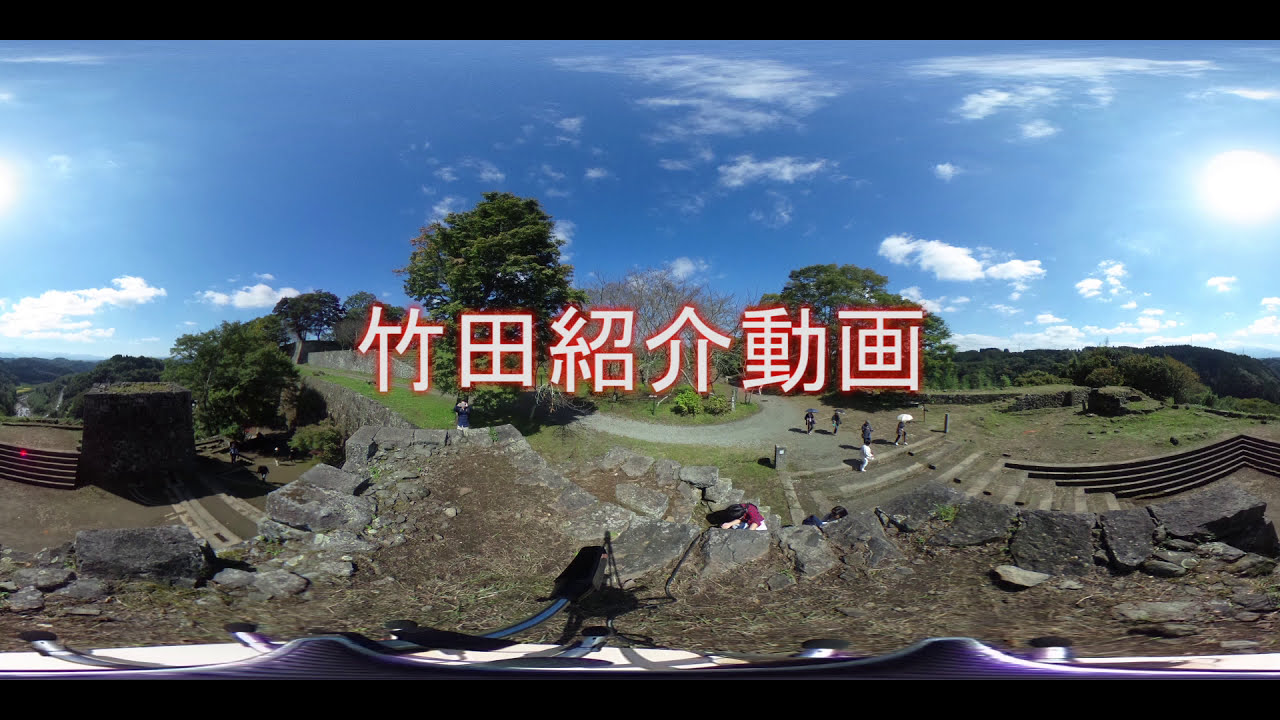In this outdoor image taken during a clear, sunny day, we see a scenic area that resembles a historical or cultural site, such as around temples commonly found in Asian countries. The focal point of the image is six white characters with an orange-red hue, most likely Chinese or Japanese, centered amidst the scene. The landscape is characterized by a rocky outcropping and hillside, with crumbling stonework that adds a touch of antiquity. On the right, stone steps descend, obscured slightly by a stone ledge. A group of five or six people, some with umbrellas likely used for sun protection, are seen walking down these steps. 

To the left, additional staircases lead to a tower area, indicating multiple levels and tiers typical of temple complexes. Some people are visible in a lower courtyard area, exploring the site. The vibrant green grass contrasts with the gray stonework, suggesting a mix of evergreens amidst leafless trees, possibly hinting at a cooler season. The backdrop features towering mountains with dense tree cover under a bright blue sky, dotted with a few clouds, and the sun shining warmly. Thin black borders frame the image at the top and bottom, and some camera effect appears to have stretched white and purple equipment across the lower border. Overall, the image portrays a beautiful, expansive cultural landmark that invites exploration and admiration.